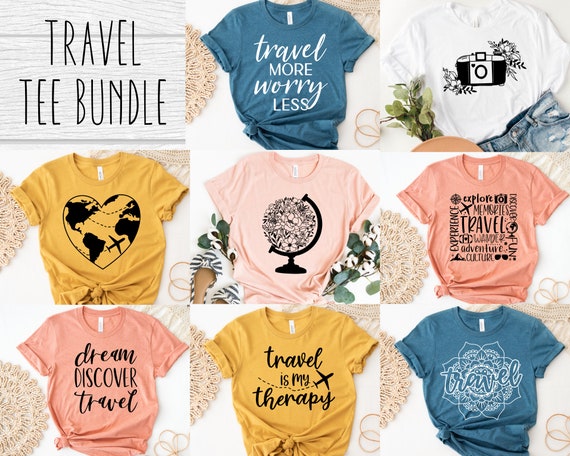This image showcases a vibrant digital poster titled "Travel T-Bundle," prominently displayed in the upper left-hand corner. The poster is a collage of eight distinct T-shirts arranged in a grid, with three rows and three columns, though the top row only has two shirts. Each T-shirt is set against a white background with subtle floral patterns. The T-shirts are in a variety of colors, including two shades of blue, light pink, mustard yellow, white, and orange.

In the top row, the first T-shirt is blue with the text "Travel More, Worry Less." Next to it, a white T-shirt displays a black camera surrounded by plants and flowers. The middle row features a mustard yellow T-shirt with the text "Travel is My Therapy" accompanied by an airplane graphic, a light pink T-shirt with a globe on a pedestal adorned with flowers, and an orange T-shirt with a word cloud containing phrases such as "Travel Memories," "Explore," "Adventure," "Culture," and "Experience," alongside images of sunglasses, a camera, and an airplane.

In the bottom row, another orange T-shirt reads, "Dream, Discover, Travel." Next to it, a light blue T-shirt displays the phrase "Travel," and the final T-shirt on the right, pink in color, features a heart-shaped globe with continents depicted in black and an airplane flying around it.

The collage’s appealing layout and the vibrant designs convey a sense of adventure, wanderlust, and the joy of discovering new places, making it an enticing visual for travel enthusiasts.